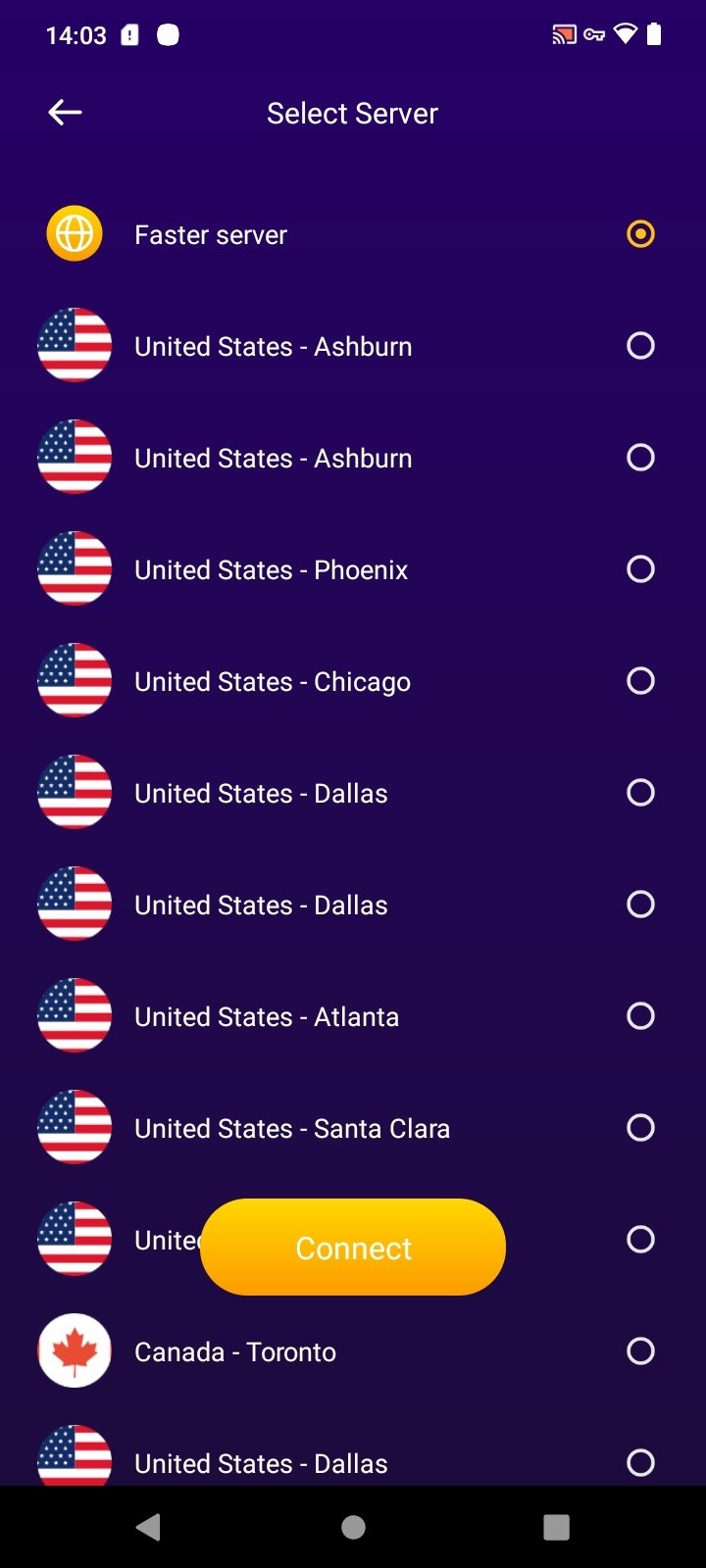The image features a predominantly purple background, with the top portion detailed and the bottom area marked as the back. On the left-hand side, a white rectangle displays the time "14:03" in white text. This rectangle has a similar color background, an exclamation point, and a light gray square.

Further elements include an outline of a white key and a white battery icon. Below these, a white arrow pointing left can be seen, situated next to the phrase "Select Server" written in white with capital S's.

An orange circle with a white globe icon appears next, labeled "Faster Server" in white text. This circle has an orange outline. Below this are various entries for server locations:
- A circle with the United States flag for multiple locations: Asheboro, Phoenix, Chicago, Dallas, Atlanta, Santa Clara.
- A circle with a Canadian flag next to the label "Canada, Toronto."

The list is interrupted by an orange oval with the word "Connecting" written in white, obscuring part of the server list. The recurring pattern involves the location name followed by a circle indicating the flag of the respective country.

This detailed visual description highlights both the functional and graphical elements present in the image.